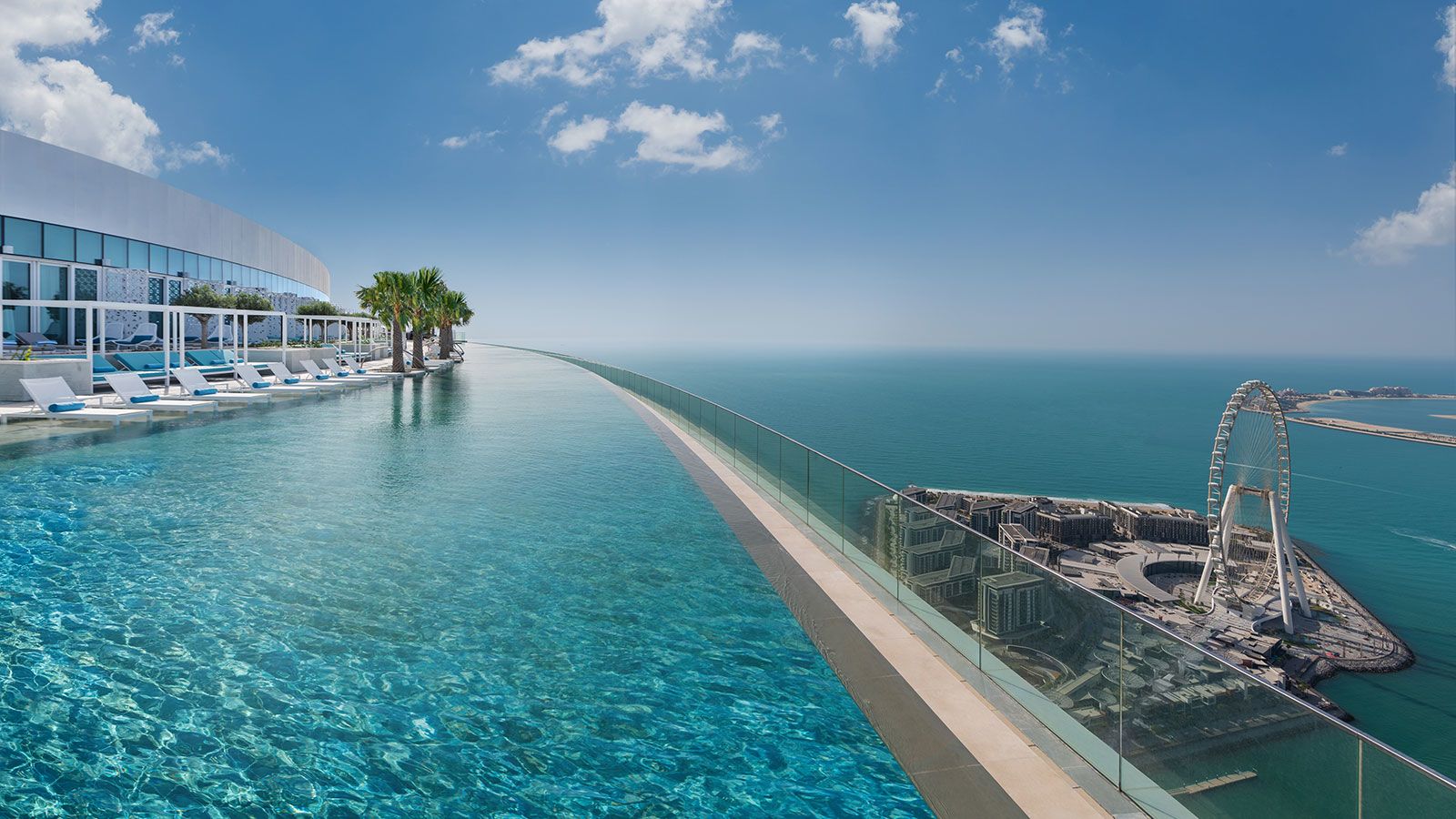The image features an opulent aerial view typical of a luxurious resort or high-end hotel. Dominating the scene is an expansive, crystal-blue infinity pool that extends towards the edge, creating a seamless view of the horizon. On the left side of the image, numerous comfortable lounge chairs are neatly arranged for guests to relax and soak up the sun under a clear, blue sky dotted with a few clouds. Adjacent to these lounge chairs, several tall palm trees and other greenery are meticulously planted in artificial soil holders, adding a touch of nature to the man-made elegance.

In the background, the sleek lines of the building's architecture are visible, featuring multiple windows and roof structures that suggest a sophisticated design. Further down, beyond the pool, a striking Ferris wheel stands, suggesting the presence of an entertainment area, possibly at a lower elevation near the base of the building. The distant view reveals a serene ocean, with a small island that hosts additional structures and the Ferris wheel, contributing to the amusement park-like ambiance. The overall composition conveys a serene yet lively atmosphere, ideal for a picturesque and memorable escape.